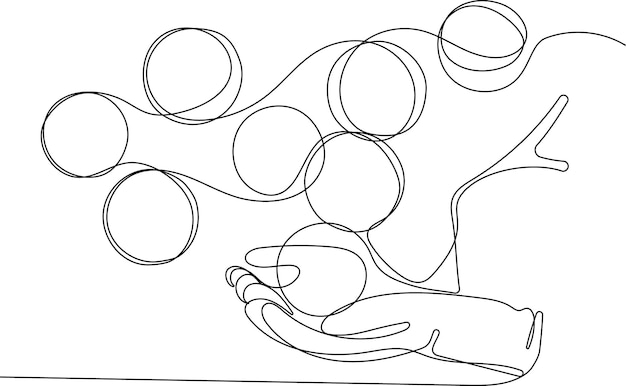The image is a minimalist black-and-white drawing composed entirely of a single, continuous, thin black line against a pure white background. The line starts from the bottom left corner and initially moves horizontally to the right before rising up to form a detailed outline of a pair of cupped hands, positioned as if ready to receive an object. Within these carefully contoured hands rests a circular shape. Extending upwards from the hands, the line continues to create a series of interconnected, swirling loops, each approximately circular. These loops, reminiscent of floating balloons or abstract orbs, are arranged in a manner that appears to defy gravity, seamlessly connected as part of the uninterrupted line. The artwork is elegant in its simplicity, combining abstract and literal elements with deliberate, fluid strokes that invite interpretation.